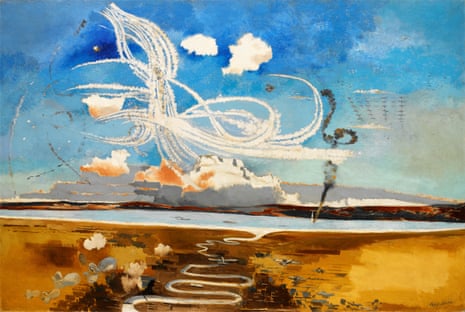This painting depicts a wartime aerial scene described in great detail. The top half showcases a serene blue sky adorned with faint, wispy white clouds. Amidst this sky, curly white contrails of swirling missiles or clusters of homing missiles paint an intricate, chaotic pattern. These curving trails lead to occasional explosions of orange hues on the horizon, suggesting distant blasts.

In the background, the blue sky features what could be interpreted as an ambiguous white figure—a man with long, cloud-like hair merging into the clouds, standing ethereal in the middle of the canvas.

The bottom half transitions into a landscape dominated by a large lake that narrows into a winding, squiggly river traveling towards the foreground. The sandy earth ground, with its brown and orange tones, is punctuated by small, dwarf-like planes parked on the brown terrain. On either side of the river, expansive yellow plains stretch out, with darker patches hinting at the battle's aftermath.

Combining elements from various perspectives, this painting fuses serene natural beauty with the ominous signs of conflict, creating a vivid and haunted wartime tableau.